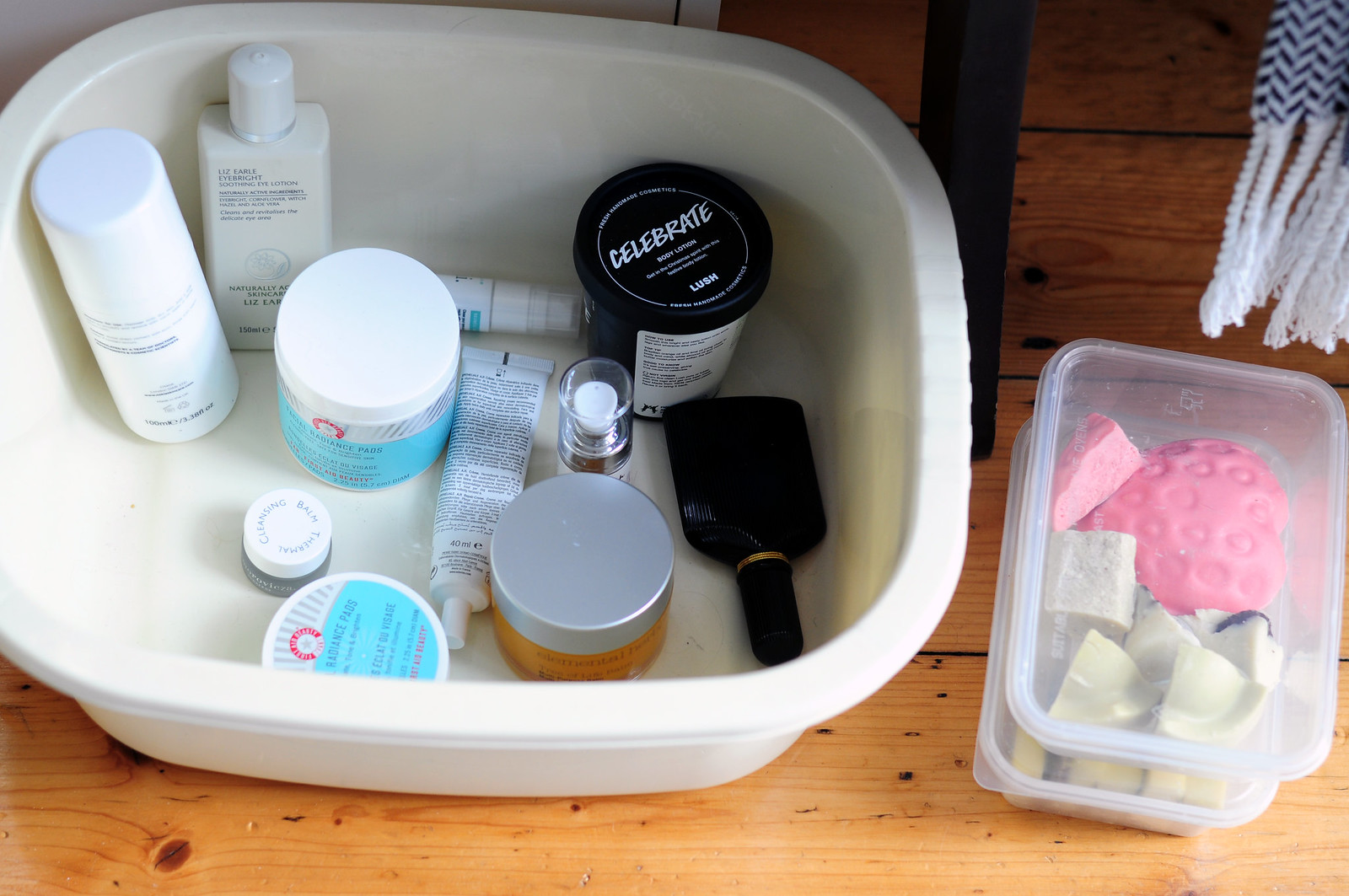This color photograph captures an oblong white plastic container that occupies much of the upper left-hand corner of the image, set against a light brown, wood-grain tabletop with darker brown streaks. The lidless container allows a clear view inside, revealing a black container labeled "CELEBRATE," which features a black lid and a white label. Next to it, a white cylindrical object stands upright, sporting a white cap and a white label with dark blue lettering. Behind it, a square, faceted canister with a smaller white cap is visible. Multiple smaller jars with white caps and light blue labels are also present, alongside a white tube with black text, its tip pointing downward.

To the right of this main container, on the same tabletop, are two stacked translucent containers with lids, through which the contents are visible. Inside, one can spot a strawberry-pink colored item, possibly soap, along with fragments of soap in various shades of pink, beige, and white.